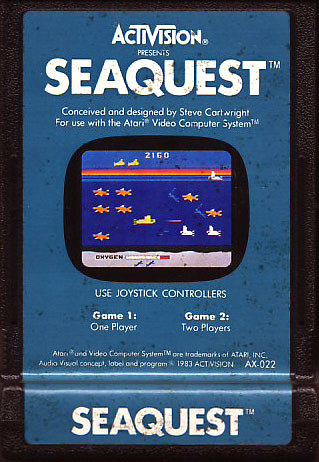This detailed image is an advertisement for an Atari video game titled "SeaQuest," presented by Activision. The advertisement has a portrait format with a black border and a blue background, highlighting white text at the top that reads "Activision presents SeaQuest." The game, conceived and designed by Steve Cartwright, is designed for use with the Atari Video Computer System. 

A central screenshot of the game showcases its vibrant underwater environment, featuring a yellow submarine navigating through blue waters, surrounded by orange fish and other marine objects, with an oxygen meter visible at the bottom of the screen. Beneath this, additional text details the gameplay options, stating "use joystick controllers, game 1: one player, game 2: two players."

Further down, there's blurred but identifiable copyright information mentioning 1983 Activision and specific product details like "AX-022." Finally, at the very bottom, the name "SeaQuest" is reiterated in white text, solidifying the game's title.